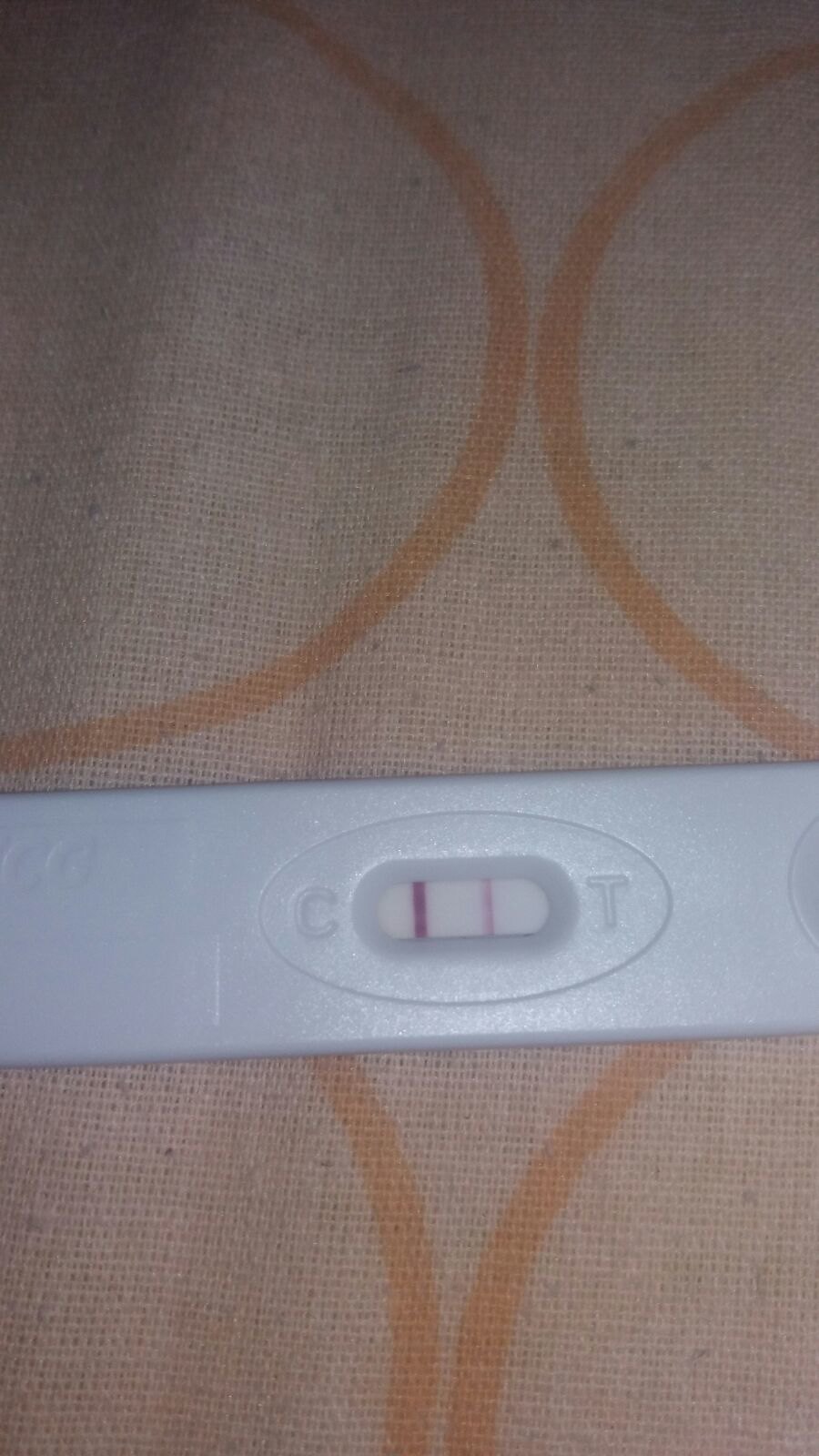This image depicts what appears to be a diagnostic test strip, commonly used for medical purposes. The test strip consists of a plastic band featuring a pill-shaped window in the center. This window showcases a sequence of colored segments: a small red segment followed by a larger white segment, a thin red segment, and then another larger white segment. The band itself is a bluish-white hue. 

On the left end of the strip, there's a letter "C," and on the right end, a letter "T," suggesting this is likely a control (C) and test (T) indicator, characteristic of tests such as pregnancy tests. The strip is placed on a burlap-like fabric background, situated between two sets of orange circular patterns, which could be either partial or half circles due to the close-up nature of the photograph. The overall setting provides a rustic texture to the image, contrasting with the clean, clinical appearance of the test strip.